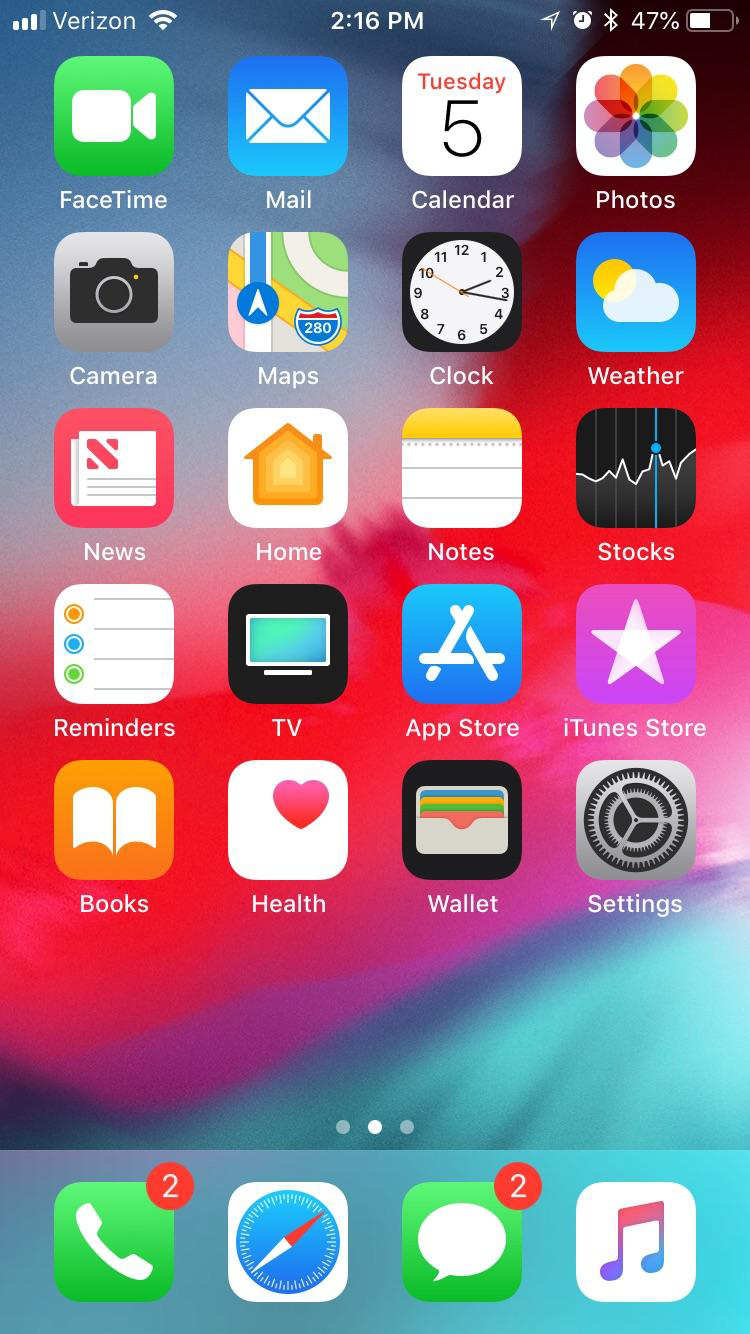This image displays a snapshot of a smartphone home screen. At the top of the screen, the status bar indicates the carrier is Verizon, with a strong signal, the time is 2:16 PM, and the battery is at 47%. The background is a vibrant, swirling gradient transitioning from blues to pinks to aquas. 

The home screen icons are neatly arranged and include:
- FaceTime
- Mail
- Calendar
- Photos
- Camera
- Maps
- Clock (depicted with an old-fashioned design featuring minute, hour, and second hands)
- Weather
- News
- Home
- Notes
- Stocks
- Books
- Health
- Wallet
- Settings

At the bottom of the screen, there's a dock with several essential apps:
- Phone (in a teal box)
- Compass
- Messages (in a green box with two unread messages)
- Music (in a white box with a musical note icon)

The overall aesthetic is both functional and visually appealing, with the colorful background enhancing the standard app icons.